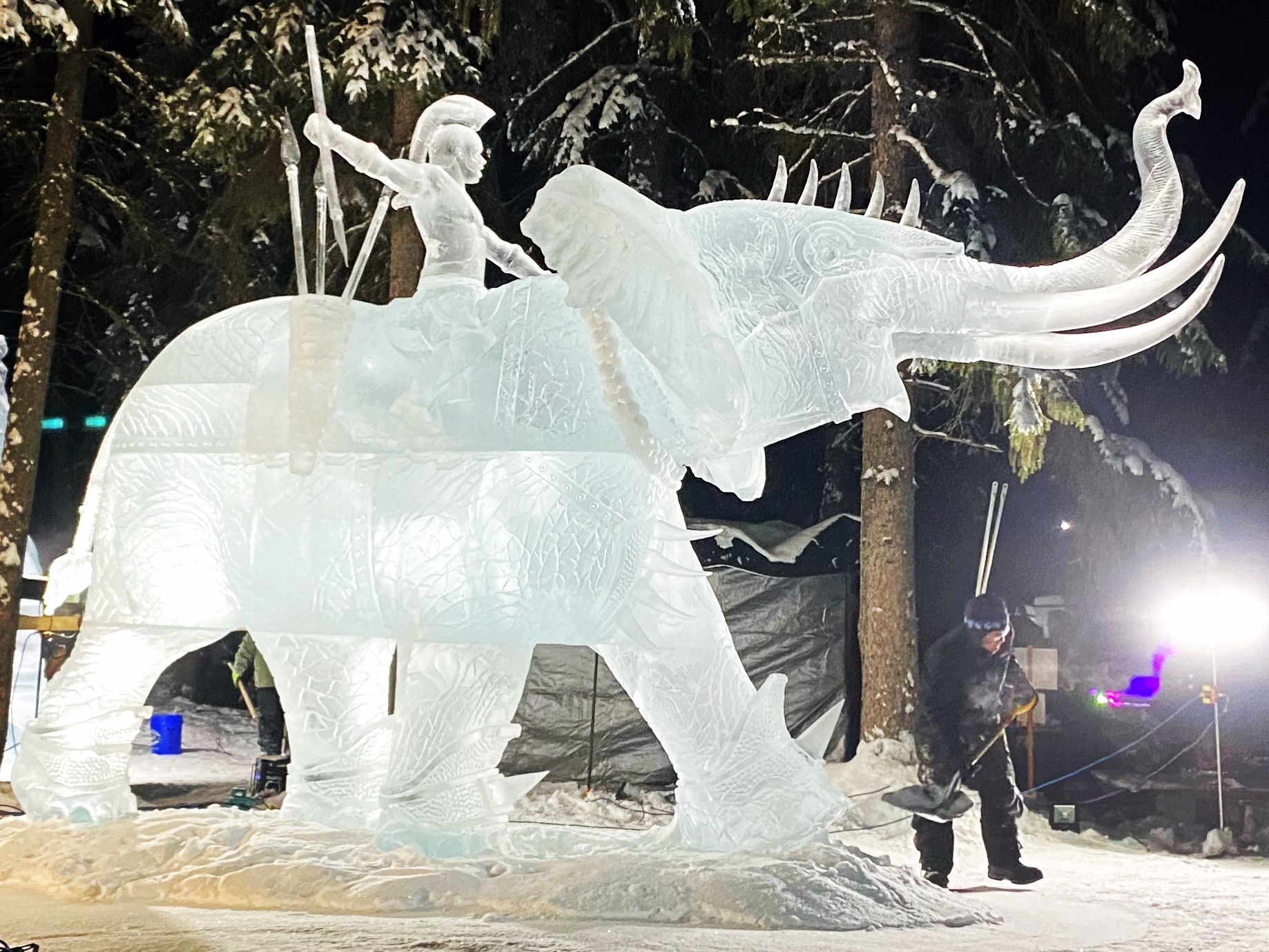In this striking nighttime photograph, a beautifully detailed ice sculpture of a majestic elephant stands as the centerpiece amidst a snowy landscape. The elephant's tusks extend forward, pointing to the right, and its trunk curls upwards as if it's blowing. Five intricate spikes protrude from its head, and its ears are splayed outward. A delicate carving creates the appearance of a necklace around its neck, and its feet are clad in spiked armor. Atop the elephant sits a knight made entirely of ice, equipped with a sword in hand and a mohawk helmet. The warrior also carries spears, javelins, and has a pouch on the side of the elephant.

Surrounding the sculpture, a thick layer of snow blankets the ground, forming a small mound beneath the elephant. In the foreground, an older man, dressed in a black snowsuit, a black hat with white accents, black boots, and wielding a black shovel, is diligently shoveling snow. He works under the bright illumination of a street lamp, which casts a glow across the scene. To the right, partially visible in green pants and jacket, another person appears to be assisting with the sculpture. Behind the elephant, trees coated in light snow stretch into the dark, starless sky, adding to the serene winter atmosphere. A blue bucket and a gray, rectangular tent can also be seen, indicating an ongoing project. This captivating image blends the artistry of ice sculpting with the quiet industriousness of snow removal, all set against a tranquil, snowy night.